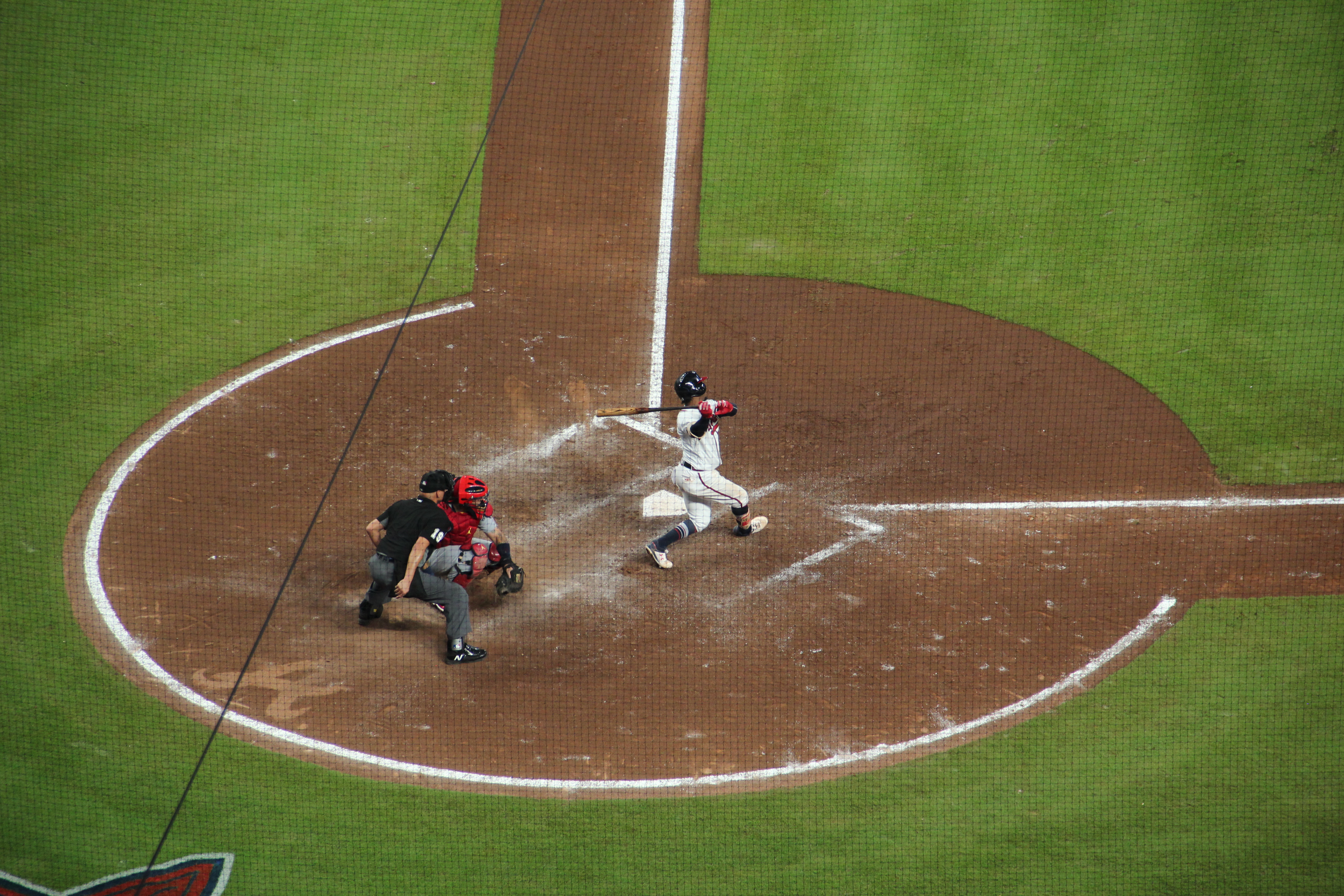In this image, we observe a vibrant scene on a large, flat grassy baseball field with a dirt infield area at its center. The photograph, captured from a moderate aerial perspective, prominently features the home plate area encircled by brown dirt. At the core of the image, we see a batter in a white uniform and dark helmet, positioned towards the upper right while swinging the bat behind him. Directly behind the batter stands a catcher, wearing a red outfit and helmet, crouched in his position. Further back is the umpire, dressed in a black top and gray pants, also crouched with bent knees overseeing the play. Surrounding the central action, the green grass of the field contrasts with the brown dirt paths leading from the home plate, indicating the base paths the batter would run. The presence of a partially visible logo in the bottom left corner suggests an official or perhaps team insignia, although it’s slightly cut off and indistinct. The setting is clearly outdoors with the activity illuminated by natural daylight, capturing a moment in what appears to be a well-maintained baseball field, ready for play. The dynamic compositions of colors including green, brown, white, red, maroon, and gray highlight the field's features and the players' uniforms, encapsulating the essence of baseball in a detailed and lively snapshot.